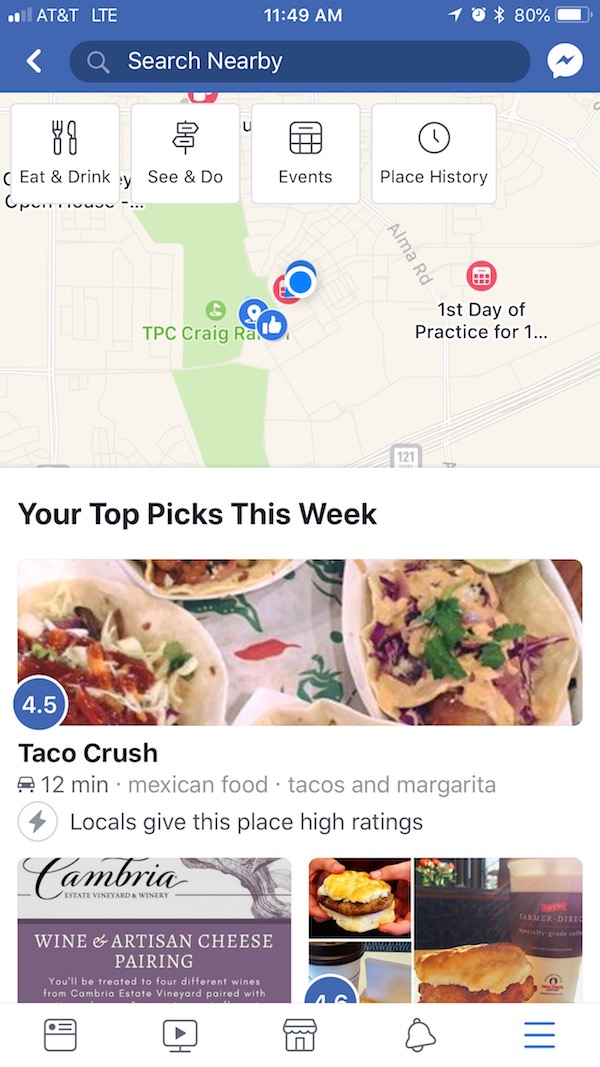The image displays a detailed screenshot from Facebook, showing a map and information about a restaurant area. At the very top, there's a blue bar, displaying the cell signal and carrier (AT&T, LTE), along with the time (11:49 a.m.). On the right, the battery percentage, alarm clock icon, and active Bluetooth icon are visible.

Below this top bar, a search bar is centered with the text "Search nearby". Next to it, on the top-right, is the Messenger icon, featuring a white speech bubble with a blue lightning bolt inside. Underneath the search bar, there are tabs labeled: "Eat and Drink," "See and Do," "Events," "Place," and "History," displayed on a beige-colored map which includes various icons marked in blue and red.

Beneath these tabs, the section "Your Top Picks This Week" highlights local attractions. First is "Taco Crush," accompanied by a tempting image of tacos. This restaurant has a 4.5 rating, is 12 minutes away by car, and is noted for its Mexican food, tacos, and margaritas, with locals giving it high ratings. Below this, there is a mention of "Cambria Estate Vineyard and Winery."